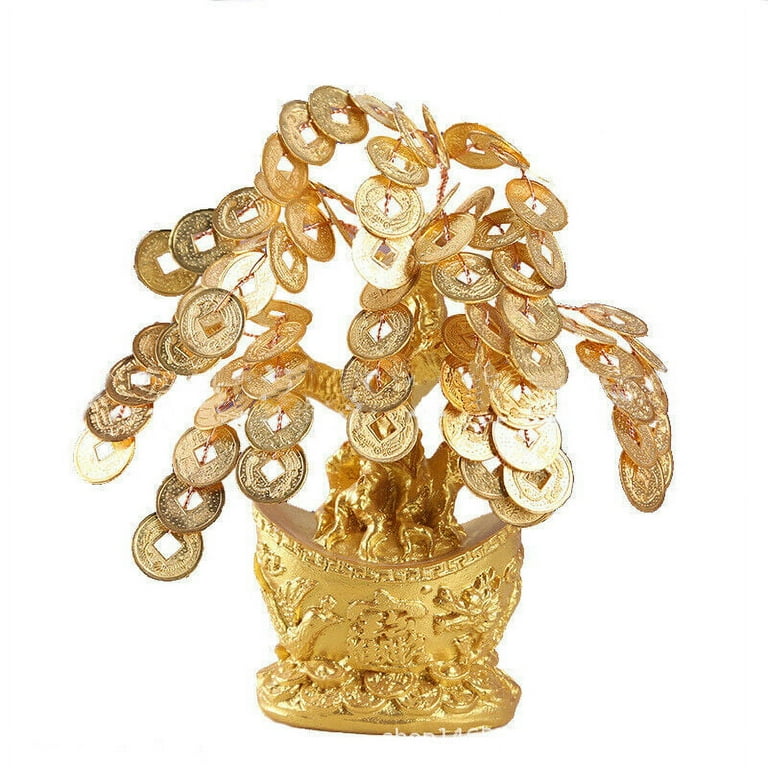In this close-up photograph, the central focus is on a lavish decorative item, designed to resemble a tree. Both the tree and its branches are intricately fashioned from golden coins, each featuring a square-shaped hole in the middle. While most of the coins maintain a bright golden hue, some exhibit a darker, tarnished quality. The trunk and branches of this metallic tree also shimmer in gold, intricately shaped to convey an aura of opulence.

The tree is anchored in an ornate, wide-mouthed golden pot that is richly decorated with elaborate designs, including what appear to be mythical creatures such as dragons or lions. The entire structure, from the pot to the tree's apex, exudes a sense of luxury and wealth, possibly symbolizing prosperity. The background of the image is a plain white, which enhances the striking golden details and gives the tree a symbolically radiant presence. Wire elements subtly support the branches, making the coins appear as if they naturally form the leaves. This artistic creation may remind one of imagery often seen on slot machines, underscoring themes of fortune and affluence.